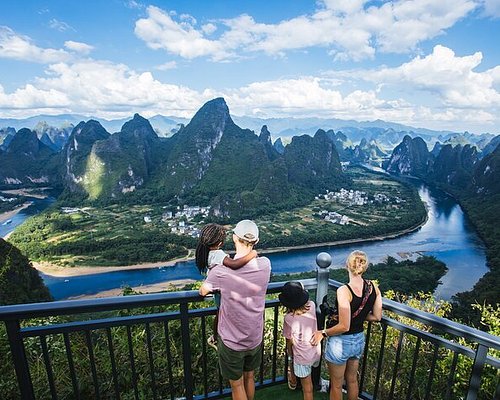A family of four is on vacation, standing on a viewing platform with a black railing, surrounded by green shrubbery. The family consists of a fair-skinned father in a pink short-sleeved shirt and green shorts, holding one of their two darker-skinned daughters, who has her arm around his neck. The fair-skinned mother, with blonde hair, is dressed in a black tank top and jean shorts, gently placing her hand on the back of their other daughter, who is wearing a black bucket cap, a pink shirt, and shorts. They are all gazing out at a breathtaking mountainous landscape, characterized by sharply craggy and tall green peaks. Below them, a blue river flows in a U-shape, encircling a lush, green island featuring a quaint village with visible houses, businesses, and a road. The viewpoint from above accentuates the picturesque setting, suggesting a location that could be reminiscent of a scenic spot in Switzerland.